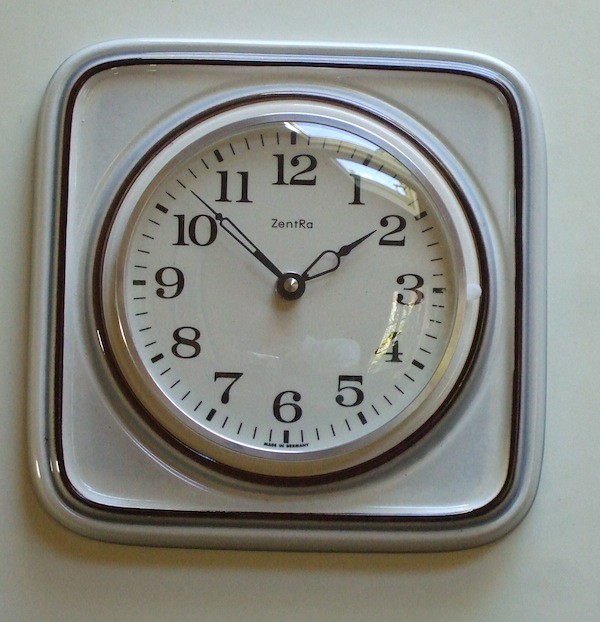This image is a detailed close-up of a clock that fills almost the entire frame, set against a pristine white background. The clock itself has a unique rounded square shape, described as having a light gray outer barrier, or perhaps a ceramic tile-like material. The central clock face is circular, off-white, and features a black outer rim. The face of the clock displays black numbers from 1 to 12 in a standard format, with bold increment lines marking every five-minute interval in between finer minute markers. The two hands of the analog clock are positioned to show the time as eight minutes to two. Above the clock hands, the brand name "Zentrah" is visible, with capitalized 'Z' and 'R'. A small shadow also appears around the bottom and slightly up the left-hand side, adding depth to the image.